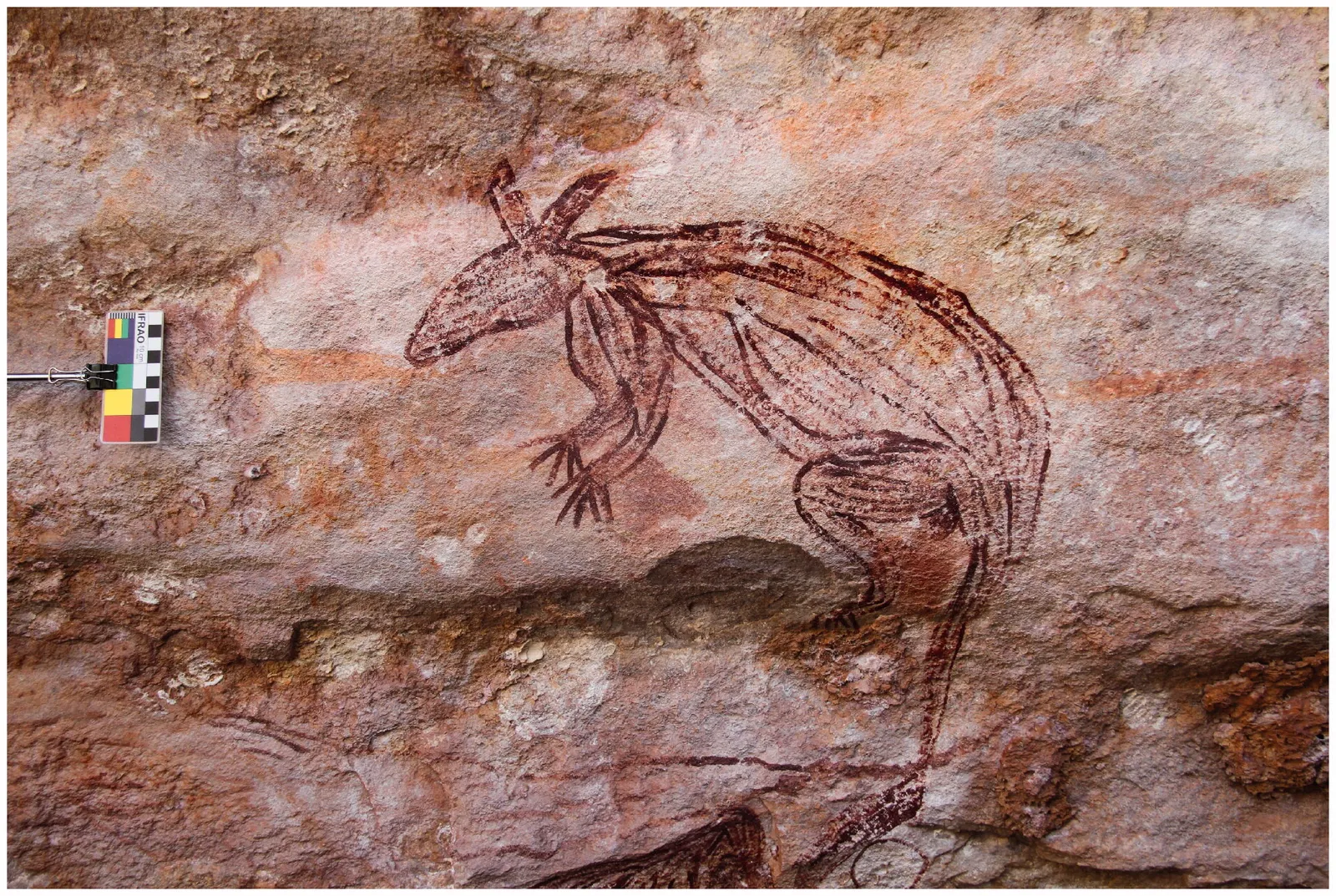This photograph captures an ancient cave drawing or engraving etched into a roughly textured stone wall, predominantly featuring a reddish-white and rust-colored palette. The artwork vividly depicts an animal poised on its haunches, which combines characteristics of various mammals. Its body resembles that of an armadillo or wombat, characterized by a long body, short forelimbs, and a long tail. The creature has an elongated snout and unusually long ears reminiscent of a rabbit’s, which contrast with its rat-like face and agile arms. This animal drawing is crudely rendered with reddish-brown markings that blend into the orange and pink hues of the stone. Additionally, there is a color gauge, possibly used in the photography process, clamped nearby for reference, providing a modern touch to this glimpse of ancient artistry.